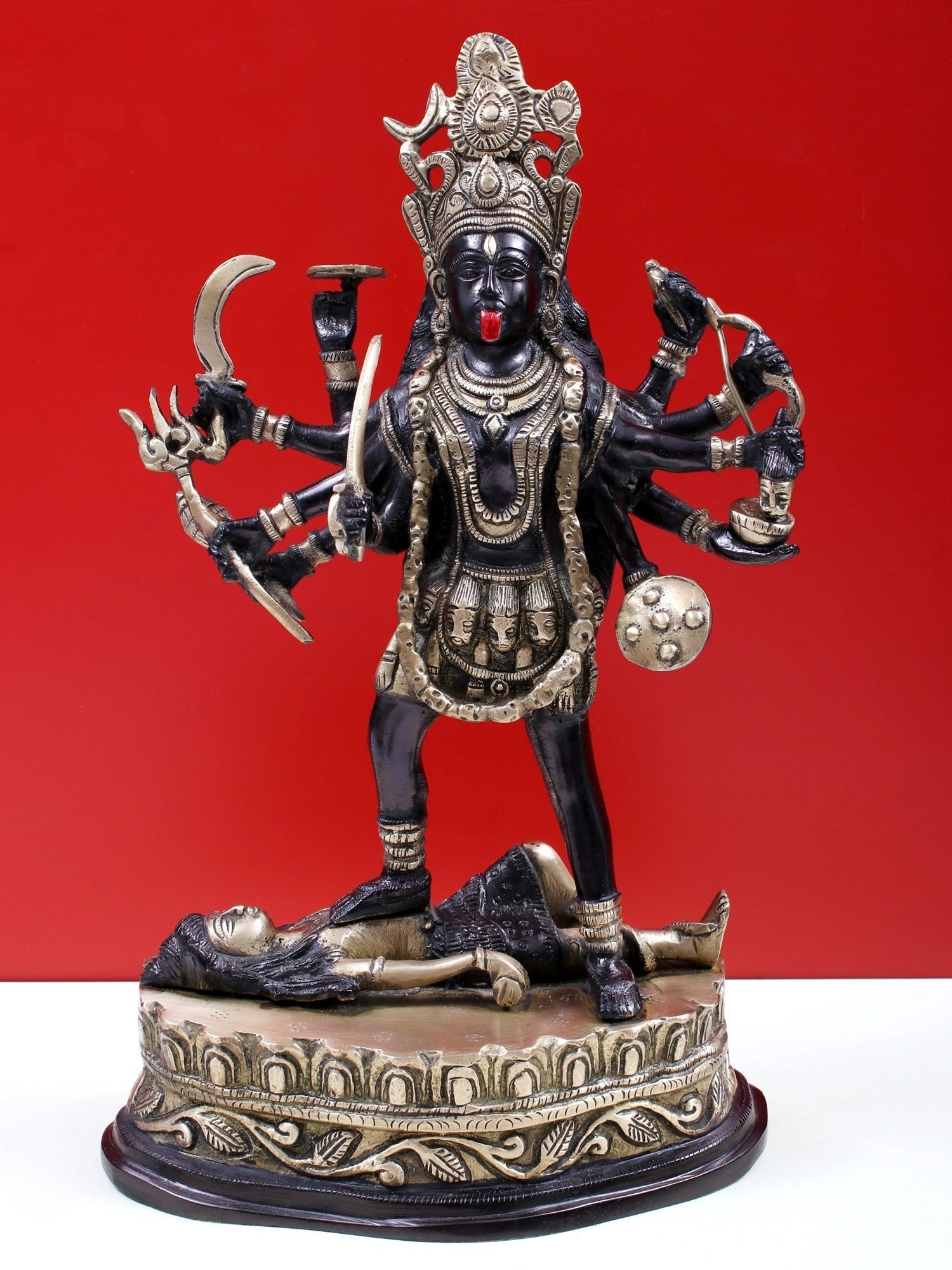The image depicts an intricate statuette of a Hindu deity, most likely representing a goddess such as Kali or Shiva, depicted with eight arms and meticulously adorned with gold and bronze jewelry. The deity, made of a black material, stands dominantly on a round base, which is ornamented with elaborate floral patterns in silver and rests on a dark bronze plinth. The deity wears an elaborate headdress and has a striking red tongue sticking out, a common attribute in representations of Kali. In each of the deity's eight hands, different symbolic items are held, including a scythe, a shield, and various weapons, showcasing the deity's powerful and multifaceted nature.

One of the deity's feet is positioned on a reclined figure of a woman, who appears lifeless with long hair, a black skirt, and a topless torso. The base on which this scene stands is richly decorated with leaf motifs, enhancing the divine and dramatic ambiance of the piece. The figurine is set against a red rectangular backdrop, which contrasts strikingly with the deity's black and gold coloration, further emphasizing its commanding and mystical presence.